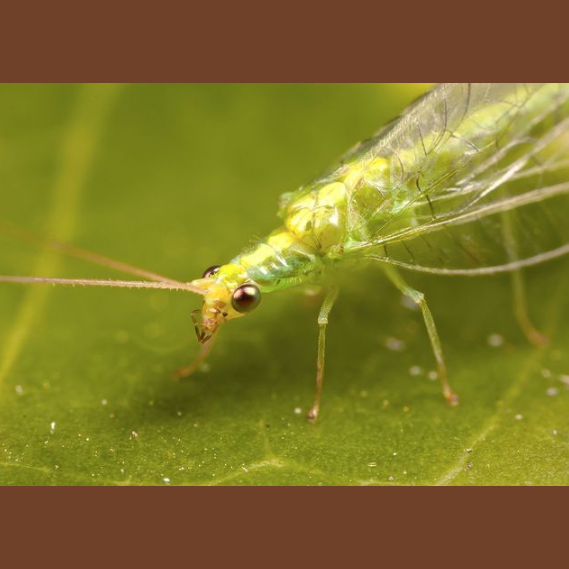This image is a very close-up shot of a green insect standing on a leaf. The insect features translucent, see-through wings detailed with visible veins, and has multiple little green legs with brown tips. Its yellowish-green head, partially see-through, houses two distinct, large, metallic-looking brown eyes that occupy a significant portion of its head. Additionally, the insect has brown antennas and pinchers protruding from its face. The leaf beneath the bug showcases a detailed texture with white veins and spots, becoming blurred towards the top of the image. The overall background is blurred, emphasizing the insect's detailed, shiny, almost semi-transparent appearance. Tan-brown banners frame the top and bottom of the image, providing contrast to the vivid green and intricate details of the insect and the leaf. The orientation of the image shows the insect’s body diagonal from the bottom left to the upper right corner, though it is cut off towards its back legs.